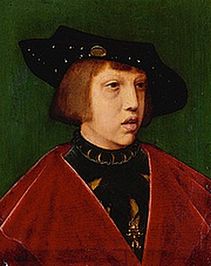A detailed Renaissance-era painting depicts a person with a distinguished appearance. The individual has short, angular, auburn hair and bangs, complementing their pale skin. They are adorned in an elegant red velvet cloak, beneath which a black top with a gold-embellished collar can be seen. A black hat, set with white studs and possibly gemstones, crowns their head. The figure's elongated nose and serious expression add to their solemn demeanor. They wear a black necklace, and the backdrop is a rich green. The person is staring off to the side, bestowing an air of contemplative mystery.